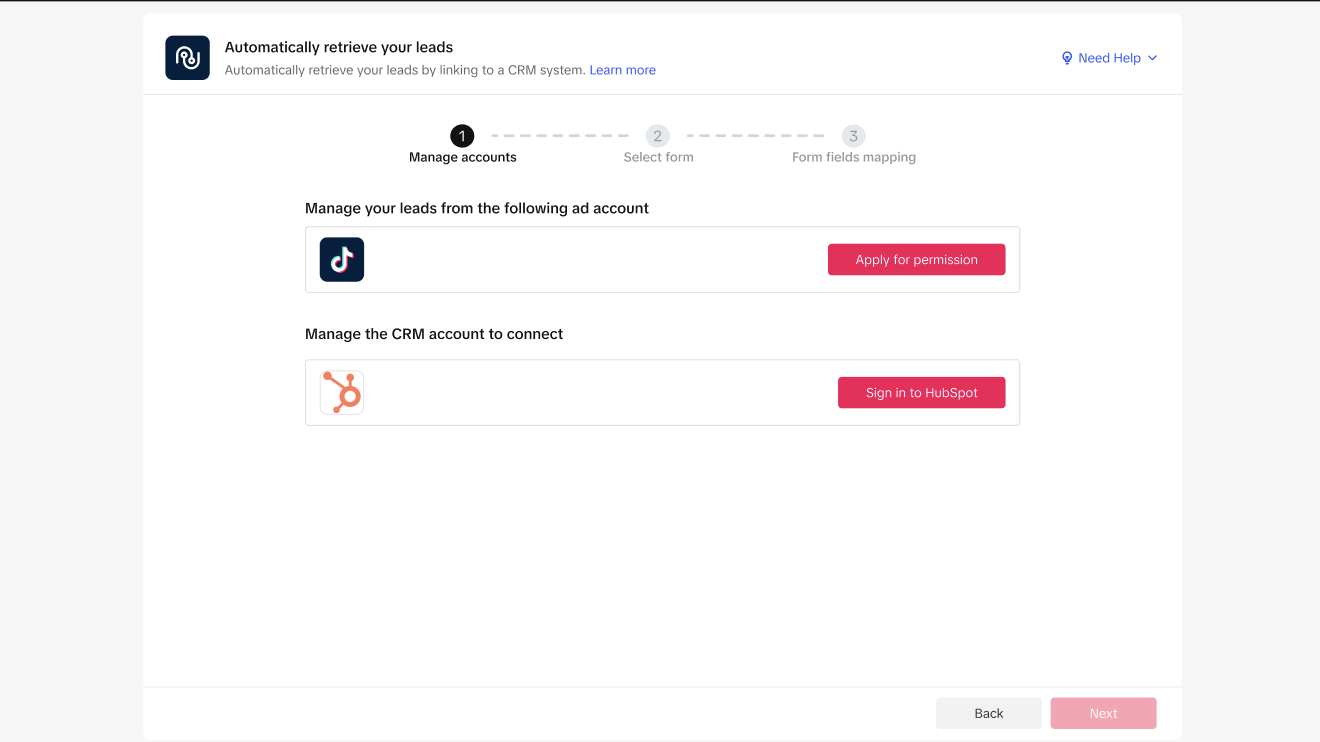The image is a left-to-right horizontal layout with a light-to-medium gray background. At the top, a thin black line runs horizontally, fading out before reaching the bottom or sides, giving it a partial border effect.

On the left side of the image, there's a small icon, either black or navy blue, adorned with a white symbol. Next to this icon, bold black text reads, "Automatically retrieve your leads." Beneath this in lighter, less bold text, it continues, "Automatically retrieve your leads by linking to a CRM system." To the right of this section, a blue hyperlink text states, "Learn more."

Towards the upper right corner of the image, another blue hyperlink reads, "Need help?" accompanied by a downward arrow, indicating a clickable element for additional assistance.

The central part of the image features a step-by-step guide. It starts with a black circle enclosing a white number "1," labeled "Manage accounts" in black text. This is followed by a series of gray dashes leading to a gray number "2" with the label "Select form," and further dashes culminating in a gray number "3" labeled "Form fields mapping." Under this progression, black text states, "Manage your leads from the following ad account." 

Below this text, there's a white rectangular box displaying a symbol resembling the TikTok logo, accompanied by an instruction in red, "Apply for permission." Further down, more black text reads, "Manage the CRM account to connect." Beside this, an orange icon is placed above a long white box labeled "Sign in to HubSpot."

At the bottom of the image, two buttons are situated: one gray labeled "Back" and one red labeled "Next."